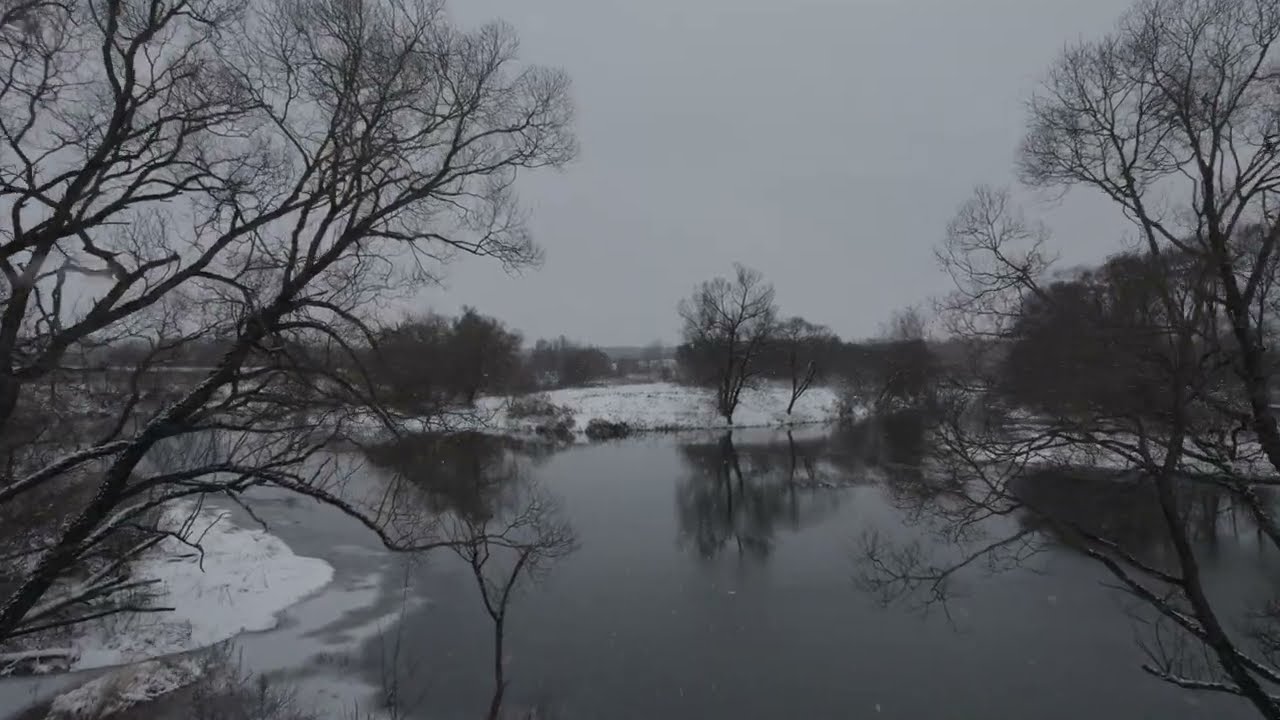This image captures a cold, bleak winter scene in nature. In the foreground, a small, frozen body of water, possibly a pond or a river, stretches from left to right, partially covered in frost. Surrounding the water, there are trees on both the left and right banks, most of which are bare, reflecting the season. The landmass at the center of the image splits the water into two streams, resembling a fork, and is covered in snow with some low bushes and one short, skinny tree emerging from it. The background features more sparse trees and faint structures that might be houses, though they are difficult to discern due to the distance and the gloomy atmosphere. The sky above is a uniform steel gray, devoid of clouds or sunlight, which adds to the overall feeling of cold and desolation. The color palette is limited to black, white, and various shades of gray, emphasizing the stark, wintry setting.